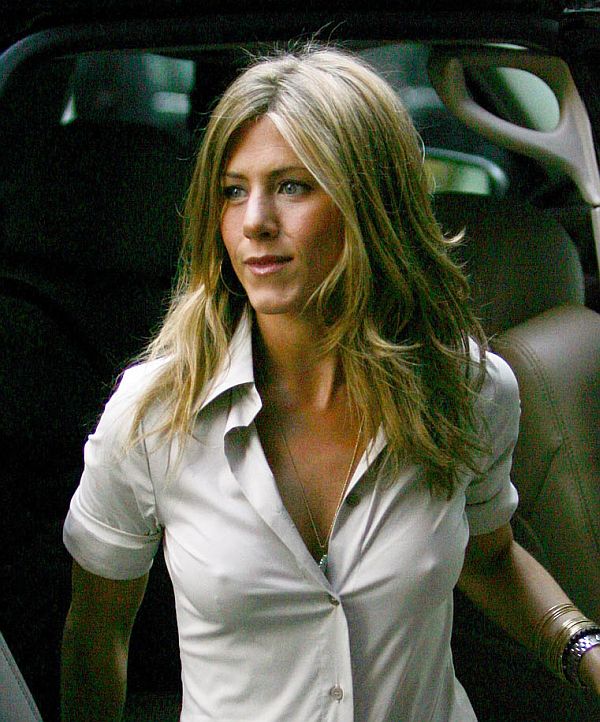This is a detailed photograph of Jennifer Aniston, captured as she is exiting a vehicle, likely an SUV or van with light tan leather upholstery. Jennifer's hair, styled long and down, is a beautiful blend of brownish-blonde and strawberry blonde. She is glancing to her right, away from the camera, with a semi-smile. 

Her attire is a casual yet stylish white button-up blouse with short sleeves that are rolled up just above her elbows, revealing numerous bracelets on her left wrist, including a stack of gold bangles and a silver watch. The blouse is open-necked, with the first button positioned between her bust, showcasing a delicate pendant on a thin chain necklace. Jennifer accessorizes her outfit with understated hoop earrings. The photograph appears to be taken during the day, likely outdoors, as suggested by the lighting filtering through the vehicle's back window.